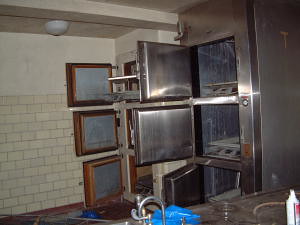The image captures a gritty and somewhat abandoned-looking industrial space. The background reveals a white brick wall that extends up three-quarters of the way, topped by a plain white section, all illuminated by a light hanging from a white edge above. Prominently, there is a large, likely stainless steel storage container on the right, featuring six open doors and an interior with blue and white panels—strongly suggesting it could be a mortuary refrigerator or cremation vault. The open doors possibly reveal pull-out gurney trays.

To the left of this container, a doorway is visible, and attached to the adjacent wall are three square panels with brown edging and white centers, aligned but slightly off-center. In the foreground, part of a grayish counter with a sink is seen, accompanied by a white spray bottle and a blue towel lying next to it. The scene is captured from a distance, adding to the overall impression of an old, maybe even abandoned space that could either be a mortuary or a kitchen, with a mix of industrial and eerie undertones.